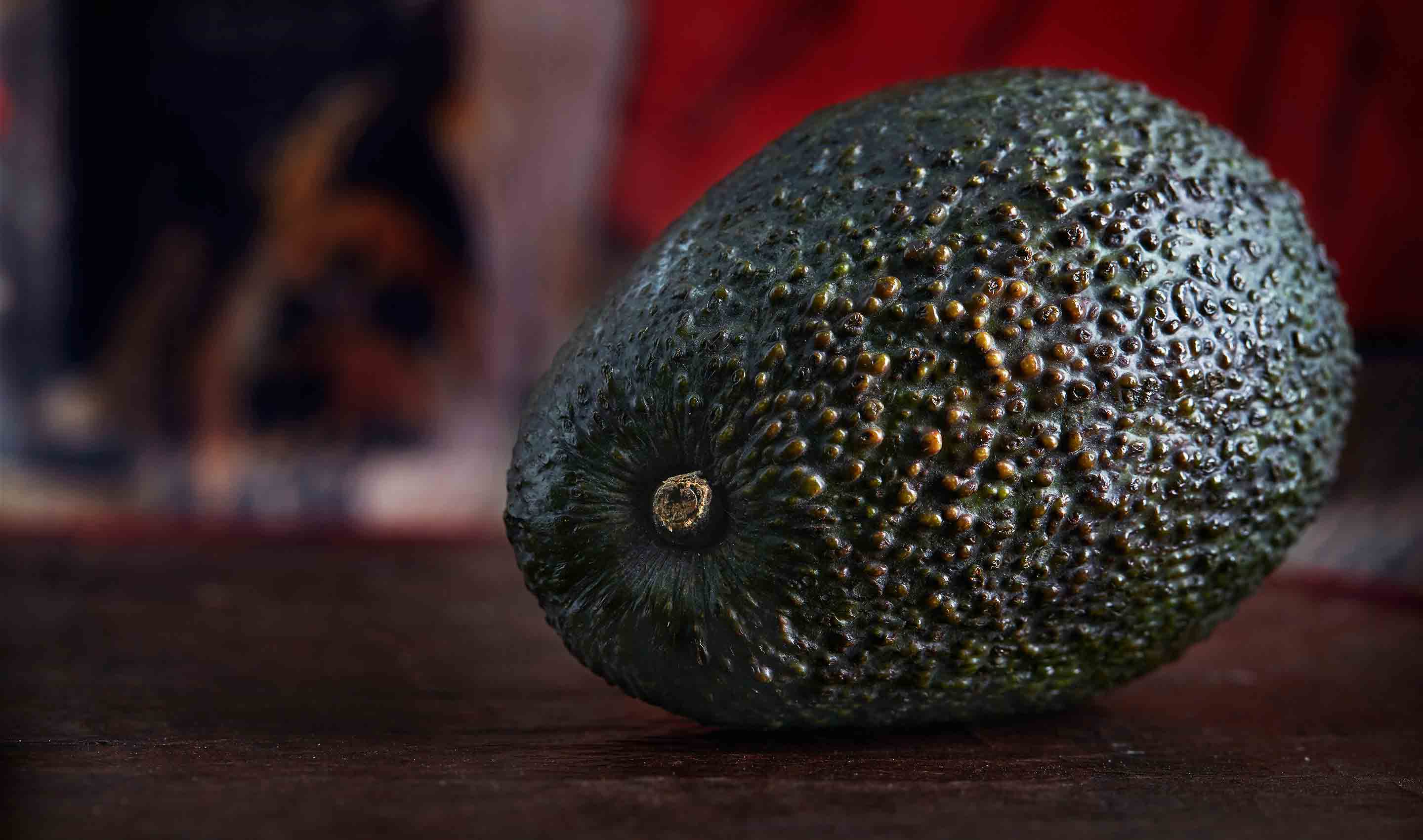The image is a close-up color photograph of a single avocado resting on a dark brown wooden surface, possibly a table. The avocado is oval-shaped and dark green, covered with numerous raised bumps and speckles, providing a rough, scaly texture. There is a small nub at the top, indicating the stub of the stem. The background of the image is blurry, featuring a portion of deep bright red, possibly a curtain or another indistinguishable object, and some darker areas, enhancing the focus on the avocado itself. The positioning shows the thinner top part of the avocado with the stem stub in the foreground, while the wider bottom part is receding into the background.